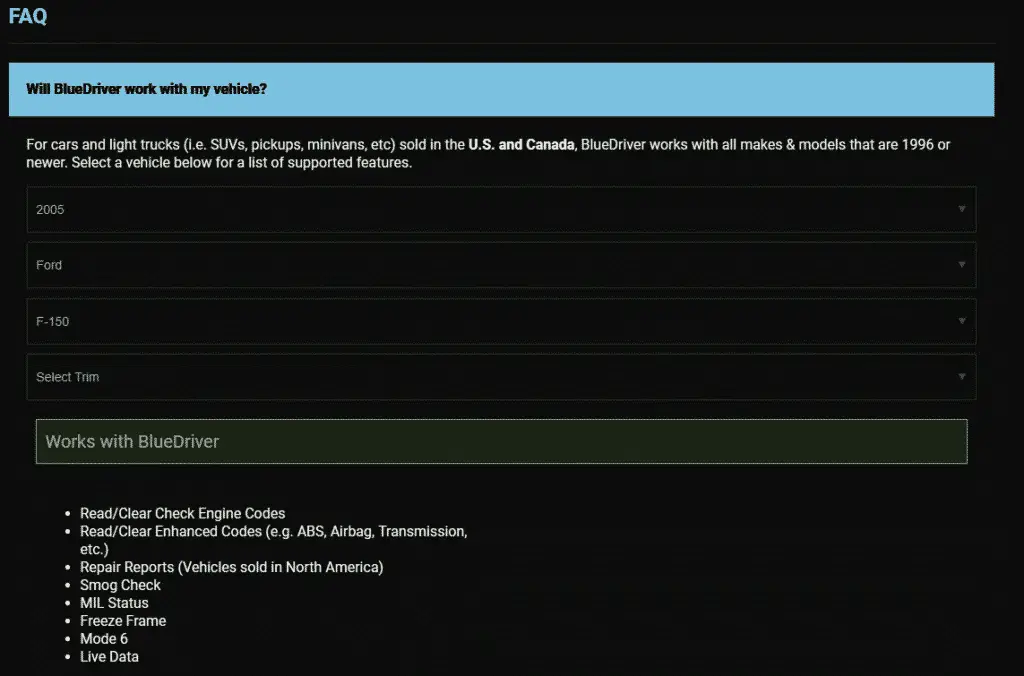The screenshot features a predominantly black background with white text concentrated at the top. At the very top, in bold blue uppercase letters, it says "FAQ." Directly beneath this, there is a small horizontal blue banner with black text that reads: "Will BlueDriver work with my vehicle?"

Underneath this banner, the following text appears in white letters: "For cars and light trucks (i.e., SUVs, pickups, minivans, etc.) sold in the US and Canada. BlueDriver works with all makes and models that are 1996 or newer. Select the vehicle below for a list of supported features."

Following this, there are four rectangular selection boxes where users can input their vehicle information. The boxes, filled in white letters, are arranged as follows: 
1. The first box reads "2005".
2. The second box reads "Ford".
3. The third box reads "F-150".
4. The fourth box, labeled "Select Trim", is yet to be filled in.

Below these selection boxes is a green rectangle containing white text that says "WORKS WITH BLUEDRIVER." Beneath this heading, there is a list of features, each prefixed with a bullet point:
- Read/Clear Check Engine Codes
- Read/Clear Enhanced Codes
- Repair Reports
- MIL Status
- Freeze Frame
- Mode 6
- Live Data